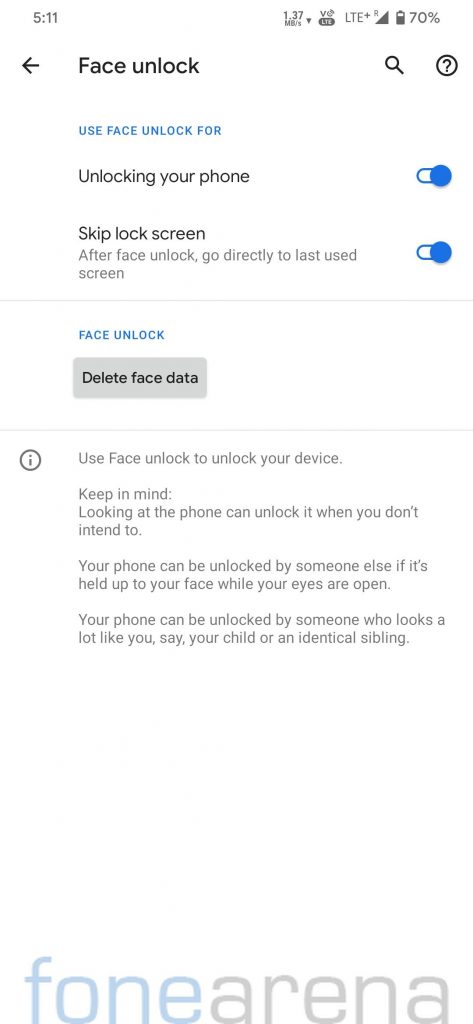The image is a smartphone screenshot showcasing the "Face Unlock" settings page from a phone application named "Fone Arena." The screenshot indicates the status bar at the top, with icons showing LTE signal strength, a service indicator, and a battery level at 70%. 

In the upper left corner, the header "Face Unlock" is displayed, with a subheading in blue text stating "Use Face Unlock for." Below this, in black text, there are options listed: "Unlocking your phone," "Skip lock screen," and "After face unlock, go directly to last used screen."

Further down the page, additional options are presented in blue text, including "Face unlock - Delete face data." Under this, an advisory notice in black text warns users about the potential security risks of using face unlock. It mentions that looking at the phone can unintentionally unlock it and that the phone can be unlocked by someone else if held up to the user's face while their eyes are open. The notice also highlights the possibility of the phone being unlocked by individuals who closely resemble the user, such as a child or an identical sibling.

The design of the app shows "Fone Arena" at the bottom, with "Fone" in light blue and "Arena" in gray. The overall look of the screenshot features a white background with text in varying shades to distinguish different sections.